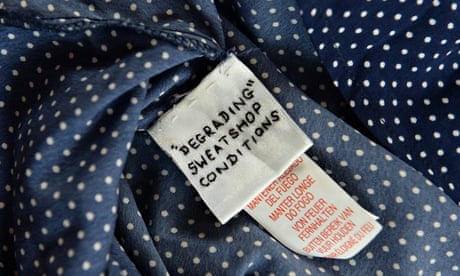This image captures the labels of a dark navy blue garment adorned with small white polka dots. The fabric appears bunched up, creating creases around the focal point: the labels. The top label is square-shaped and white, featuring black, all-caps handwriting that reads “DEGRADING” at the top and “SWEATSHOP CONDITIONS” below it. The text is enclosed in double quotation marks. This label is prominently positioned above another long, thin, rectangular label displaying instructions or information in various foreign languages in red, capitalized font. The top label appears to be hand-stitched and is attached along a seam of the garment, which could be a shirt, dress, or blouse.